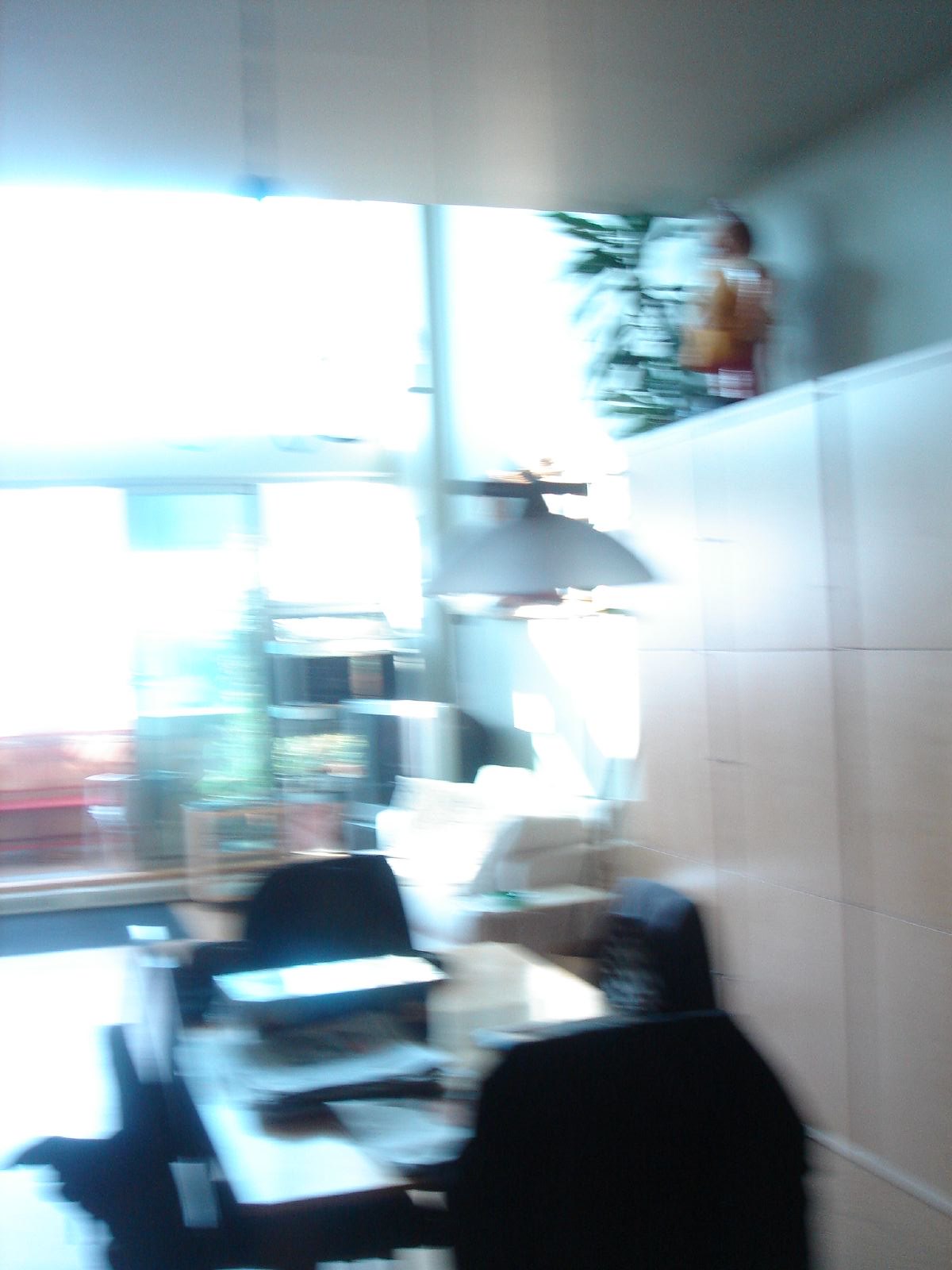A brightly lit room with expansive windows lining the back wall captures a warm, inviting atmosphere in this motion-blurred photograph. Near the right side, a wooden cabinet adorned with a decorative doll stands in front of lush green plants, adding a touch of charm to the space. In the middle of the room, two black chairs flank a central coffee table, crafting a cozy seating area. Hanging from the ceiling is a contemporary gray lamp, casting an ambient glow. Towards the rear, a white chair complements the shelves that display various knick-knacks, further enhancing the room's character and making it a multifaceted space for relaxation and decor. Despite the blur, the overall coziness and design elements are evident.